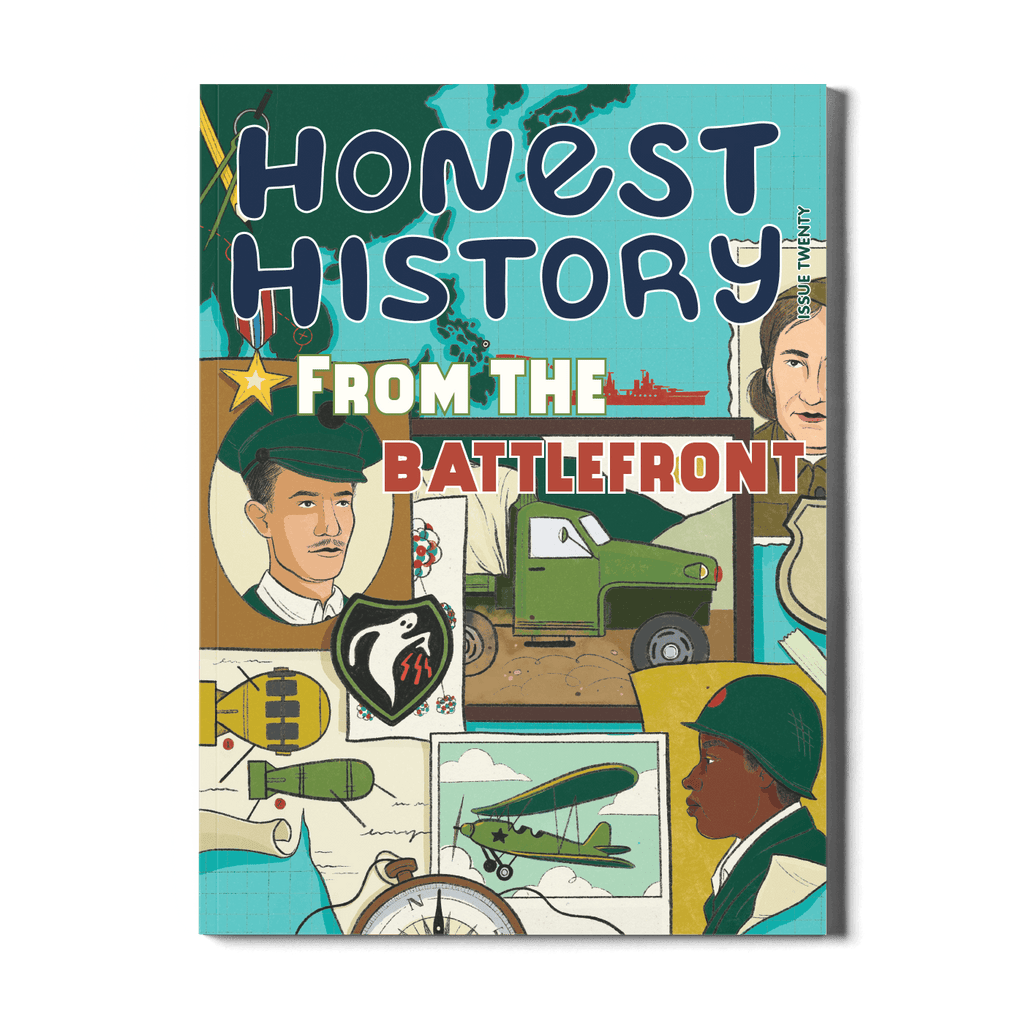The cover of "Honest History: From the Battlefront" (Issue 20) is a vibrant and intricate illustration that captures various military elements rooted in historical conflicts. The title, "HONEST HISTORY," is prominently displayed in dark blue cartoonish all-caps text, with the subtitle "From the Battlefront" in white and bold red text, accompanied by a gold star beside it. 

The background is a detailed depiction of East Asia on a world map, with turquoise oceans and dark green landmasses. Superimposed on the map are several illustrations representing different battlefront aspects. On the right side is an older woman in a nurse’s military uniform, and on the left, an officer in uniform with a green hat and thin mustache. Central to the image is a green military truck, beneath which is an emblem featuring a ghost with red lightning bolts in its hands.

To the bottom right stands an African-American soldier in a green uniform and helmet with a red circle, wearing a white-collared shirt and green vest, looking to the left. The cover also features a green biplane with a black star in the center, green and yellow missiles in the corner, and a compass at the bottom, partially covered by light blue and cream-colored triangles. The top left corner has a dark green background adorned with a pencil and a dark blue "H," while the top right corner is lighter with grid lines and crosses. The magazine highlights the contributions of people of color in military history, reflected in its detailed artwork and vivid colors.